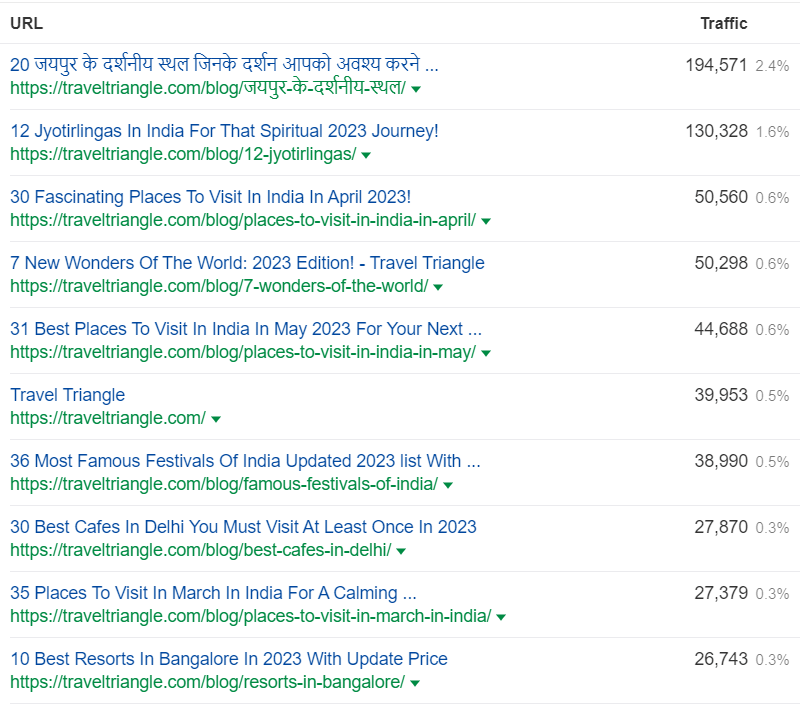This image displays traffic statistics for various URLs, primarily related to travel and destinations in India. On the left side, the titles of the websites are highlighted in blue, with the corresponding URLs beneath them in green. Each URL title seems to focus on travel-related content, such as "30 Fascinating Places to Visit in India in April 2023" and "30 Most Famous Festivals of India - Updated 2023 List." Overall, there are 10 distinct URLs listed. 

The right side of the image presents traffic numbers, detailing how frequently each site is visited. The statistics are as follows, ranked from highest to lowest traffic:
1. 194,571 visits (2.4%)
2. 130,328 visits (1.6%)
3. 50,560 visits (0.6%)
4. 50,298 visits (0.6%)
5. 44,688 visits (0.6%)
6. 39,953 visits (0.5%)
7. 38,990 visits (0.5%)
8. 27,870 visits (0.3%)
9. 27,379 visits (0.3%)
10. 26,743 visits (0.3%)

This detailed breakdown provides insights into the popularity of these travel-related websites, showcasing user engagement with content about traveling in India.